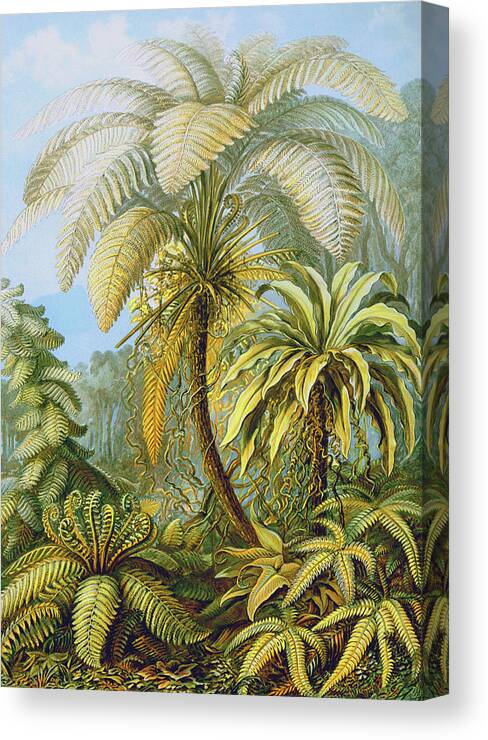The image is an oil painting on canvas featuring a vibrant and lush tropical landscape dominated by two prominent palm trees. The central palm tree, with its tall, lean trunk and large, light green to yellowish leaves, immediately captures attention. Surrounding this focal point is a smaller palm tree to the right, about half the size, with similarly colored but more wrinkled leaves. The background showcases a blue sky with a few white clouds and a dense forest partially obscured by the large palm tree. At the bottom, diverse vegetation includes clusters of ferns and various bushes, contributing to the overall richness and depth of the scene. The composition is detailed with the ground adorned with scattered leaves, enhancing the vivid portrayal of this tropical paradise.